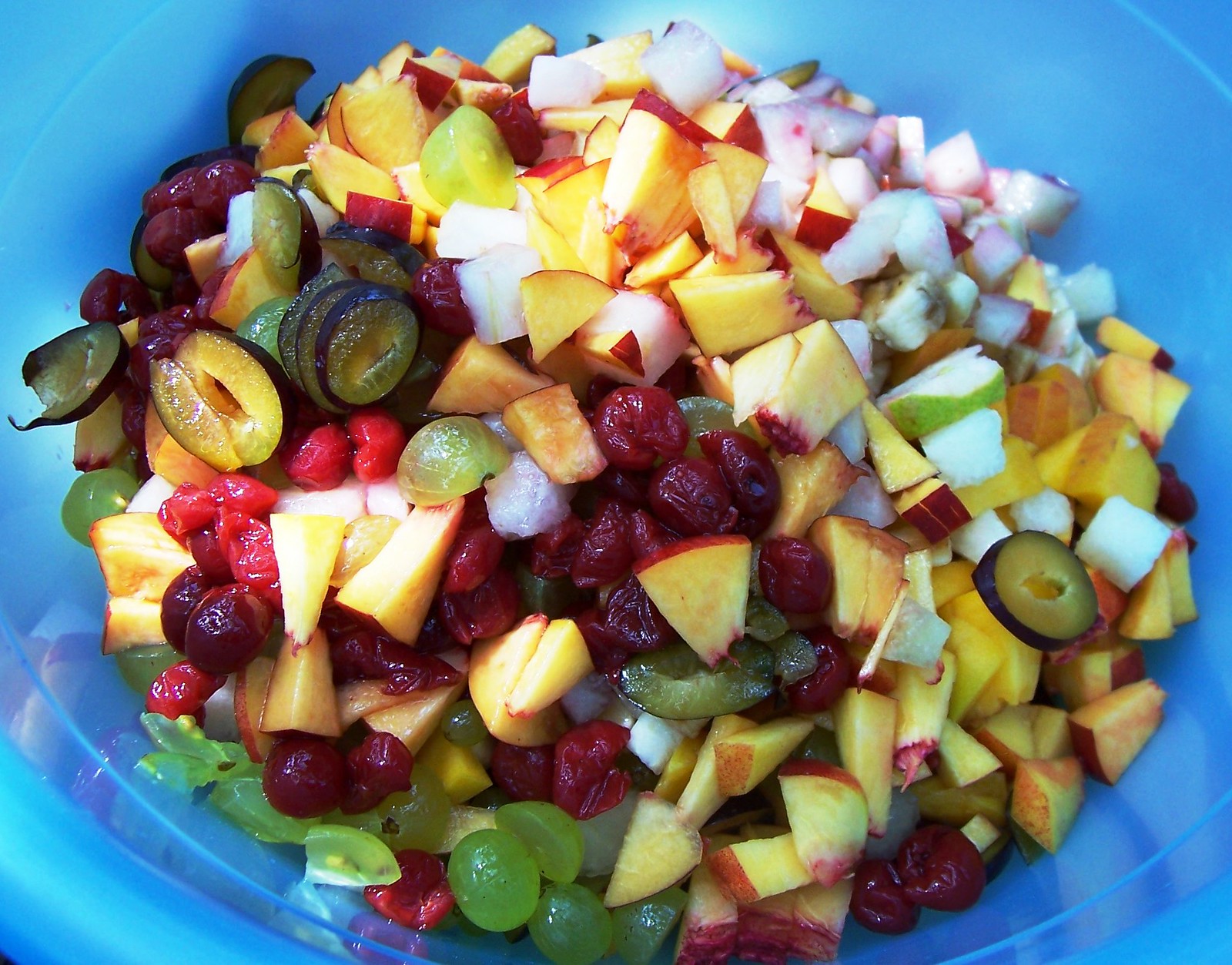The photograph captures a large blue-tinted glass bowl overflowing with a colorful and varied fruit salad that stretches beyond the frame. The bowl itself is prominent, with edges extending off the photograph, preventing any background from being visible. The fruit salad contains an array of vibrant ingredients including diced peaches, green apples, red-skinned fruits, and an assortment of grapes, some whole and some halved, in shades of green and burgundy red. Additionally, there are components in yellow, red, white, orange, and dark reddish-purple hues, contributing to the mosaic of colors and textures. Within this close-up shot, certain pieces are diced finely while others are larger, providing a rich texture variety. The detailed mix also shows tiny tomatoes, cranberries, possibly sliced olives, and hints of chopped celery and onions, making it an intricate blend of fruits and vegetables. The arrangement appears meticulously detailed, as if crafted by AI, creating an almost surreal, richly detailed depiction of a fruit and vegetable salad.